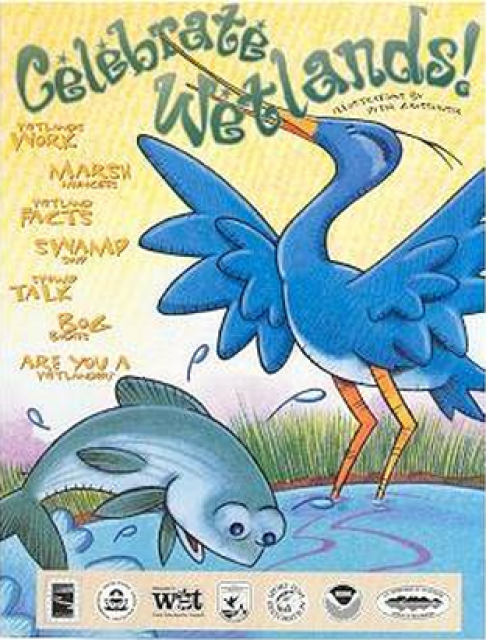This image is the cover of a whimsical children's book titled "Celebrate Wetlands!" featuring a vibrant, cartoonish design. The background showcases a yellow sky with horizontal stripes, interspersed with purple and white hues, along with patches of grass encircling a small pond. In the pond, a cheerful green fish with a light blue belly and big eyes leaps out of the water, displaying a wide smile. Beside the fish stands an elegantly illustrated blue bird, resembling a crane or heron, with orange legs, outstretched wings, and an elongated beak that whimsically intertwines with the letters of the title. Surrounding the scene, additional text in a playful font reads "Marsh, Fax, Swamped, Talk, Bog, and Are You a Wetlander?" Various logos of organizations dedicated to wetland preservation are placed at the bottom, though they appear somewhat blurry and difficult to discern.